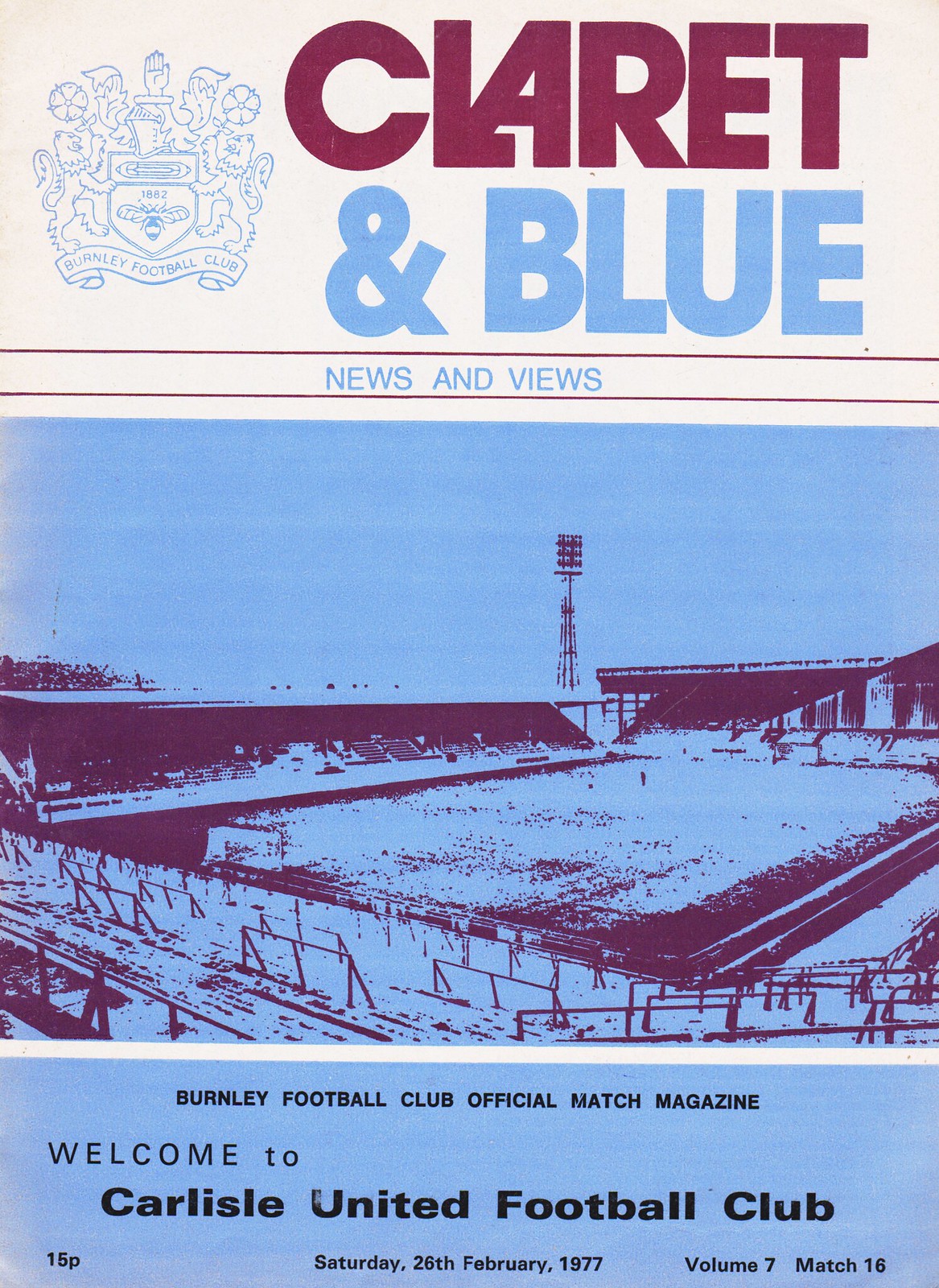The image displays the cover of a digital screenshot for a sports periodical, specifically a game day program for Burnley Football Club. The top third of the cover features a white background with text and a logo, which includes a royal seal or insignia on the left. Adjacent to the seal, the text "Claret & Blue" is written, with "Claret" in purple and "& Blue" in blue. Beneath this title, "News and Views" is inscribed in light blue within two purple horizontal lines. Centered on the cover is a monochrome blue photograph of a large football stadium, viewed from the stands. The footer of the cover has a light blue background with black text, stating "Burnley Football Club Official Match Magazine," as well as "Welcome to Carlisle United Football Club." Additional details include the price, "15p," the date, "Saturday, 26 February 1977," and publication specifics, "Volume 7, Match 16." The overall color scheme incorporates shades of blue and burgundy.